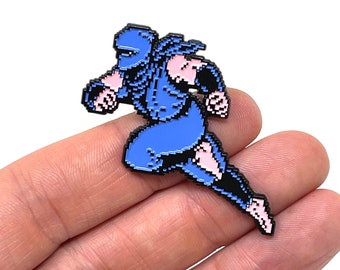In the image, three white-skinned fingers delicately hold a small, pixelated figure, possibly a pin or a tiny action figure measuring around five or six inches. The figure resembles a ninja from the video game Ninja Gaiden, dressed predominantly in blue. The ninja's outfit consists of a blue head covering that leaves only the eyes visible, a blue neckerchief flowing behind, a blue jersey with black buttons, and matching blue pants. The ninja has bulky biceps, black wrist wrappings, and boasts a dynamic pose: the right arm is crossed in front as if in a running motion, while the left arm is positioned to the side, preparing to strike or pounce. The right leg is grounded, and the left leg is lifted towards the buttocks. Notably, the character is barefoot, adding to the dynamic, action-oriented stance. The figure's intricate details, from the color scheme to the pose, highlight its vigorous, battle-ready demeanor.